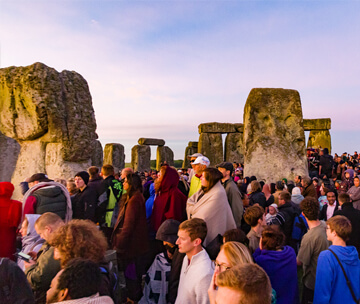This photograph captures a side view of a large crowd, likely numbering over a hundred people, gathered at Stonehenge. The individuals span multiple backgrounds, predominantly white, and are dressed in various warm clothing, indicating a chilly day. Visible attire includes hoodies, jackets, blankets, sweatshirts in colors such as brown, red, white, yellow, green, beige, and blue, and notably, a woman draped in a light blue blanket and a man in a distinctive red hoodie with a red beard. The group is densely packed within the iconic stone structure of Stonehenge, characterized by its massive, man-made stone slabs arranged in a doorway-like formation. The photo's backdrop includes a mostly cloudy sky with hints of light blue and the distant sea, while the foreground features a few individuals looking at their phones.